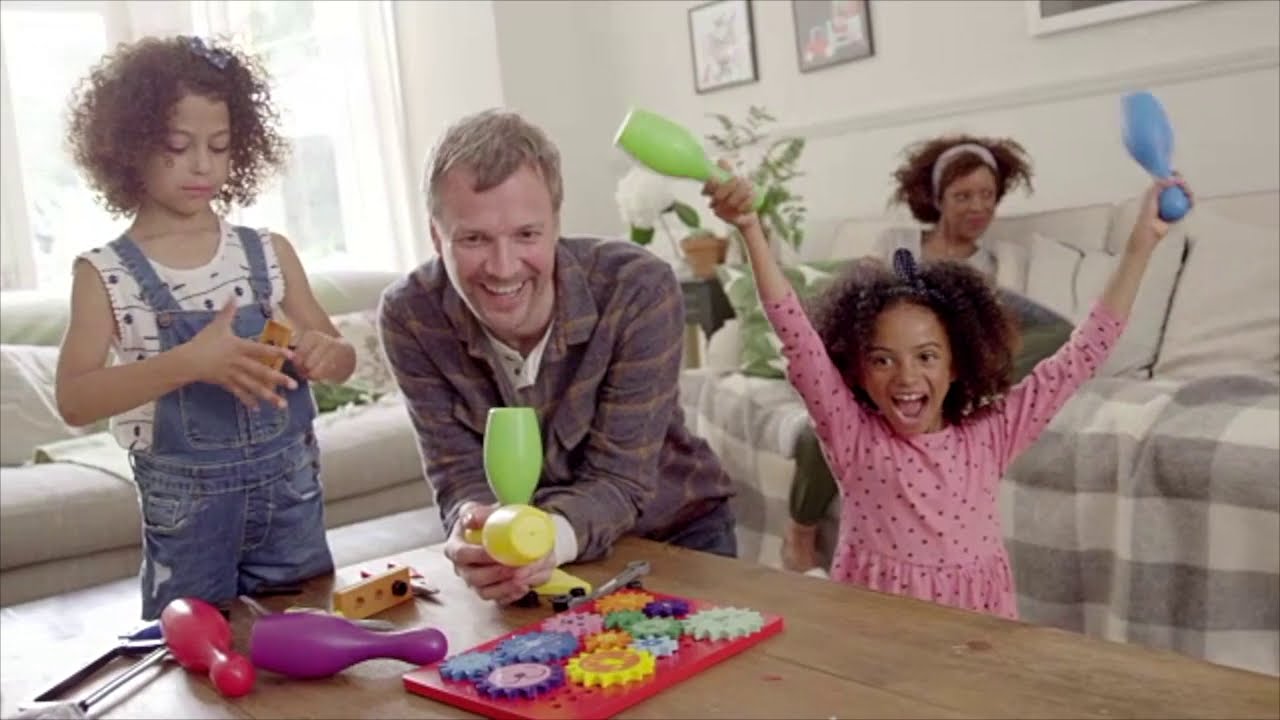In the living room of a cozy home, bathed in natural light from a large window, a family of four is gathered around a wooden coffee table. The father, a man with gray hair and a warm smile, is dressed in a purple long-sleeved shirt and is enthusiastically engaging in a board game characterized by multicolored mechanical gears and bright bowling pins. To his right, his younger daughter, dressed in a pink long-sleeved dress adorned with black polka dots, clutches blue and green bowling pins, her face lit with the joy of the game. On his left, his older daughter, sporting blue denim overalls over a white shirt, is deeply focused on a block in her hands, her curly hair framing her concentrated expression. Behind them, on one of two gray-hued couches, the mother, wearing a headband and a checkered gray and white blanket, sits watching, slightly disengaged but content, completing the picture of a serene family moment.